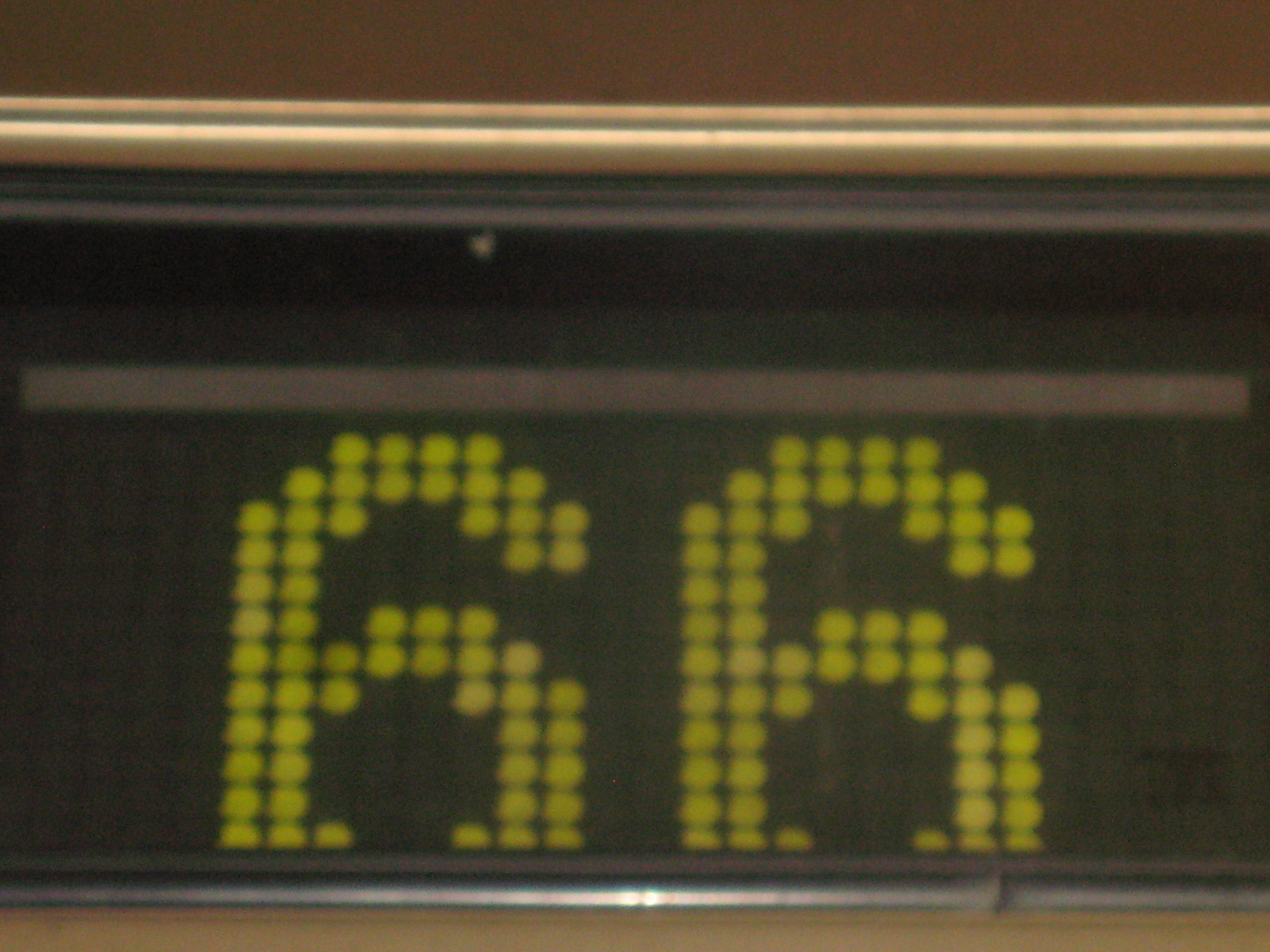This photograph captures an illuminated dot matrix display set into a wall, likely an elevator display. The display features vibrant yellow digits reading "6666" against a black background, which stands out prominently due to the bright lighting. The display is encased in a black frame, which is itself bordered by an off-white or white frame, providing a stark contrast against the brownish wall surrounding it. The angle of the photograph suggests that the display is positioned above the photographer, as the bottom part of the display is slightly cut off. The setting appears to be indoors, contributing to the controlled lighting and clear visibility of the display.